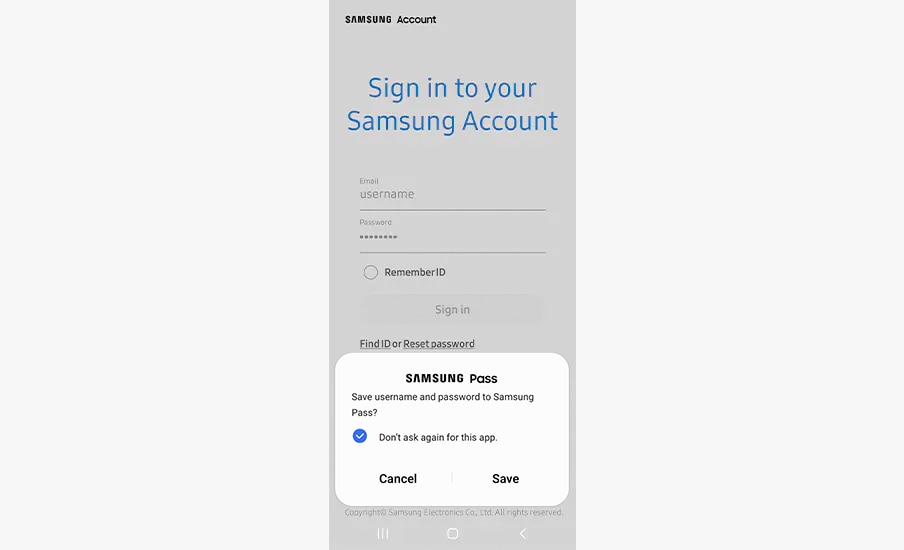The image depicts a Samsung account sign-in page as viewed on a mobile device, likely an iPhone, given the recognizable icons at the bottom of the screen. The narrow layout and consistent gray background suggest this is indeed a screenshot from a phone. The header, "Sign into your Samsung account," is prominently displayed in blue text. 

Below the header, there are fields for entering your email or username and your password, both of which are filled in this example. Just beneath these fields, there's an option to "Remember ID," which can be toggled on or off.

Further down, a gray sign-in button blends into the gray background, maintaining the overall monochromatic color scheme. Additional options such as "Find ID" or "Reset password" are also available.

A white pop-up box has appeared on the screen, featuring "Samsung Pass" at the top. This pop-up prompts users to save their username and password to Samsung Pass, with an option labeled "Don't ask again for this app," which is selected with a blue circle containing a white check mark. At the bottom of the pop-up, there are "Cancel" and "Save" buttons for user interaction, allowing them to either discard these options or save their credentials, respectively.

The presence of iPhone interface elements at the bottom of the screen, such as the familiar icons, further confirms that this screenshot was taken on an iPhone.